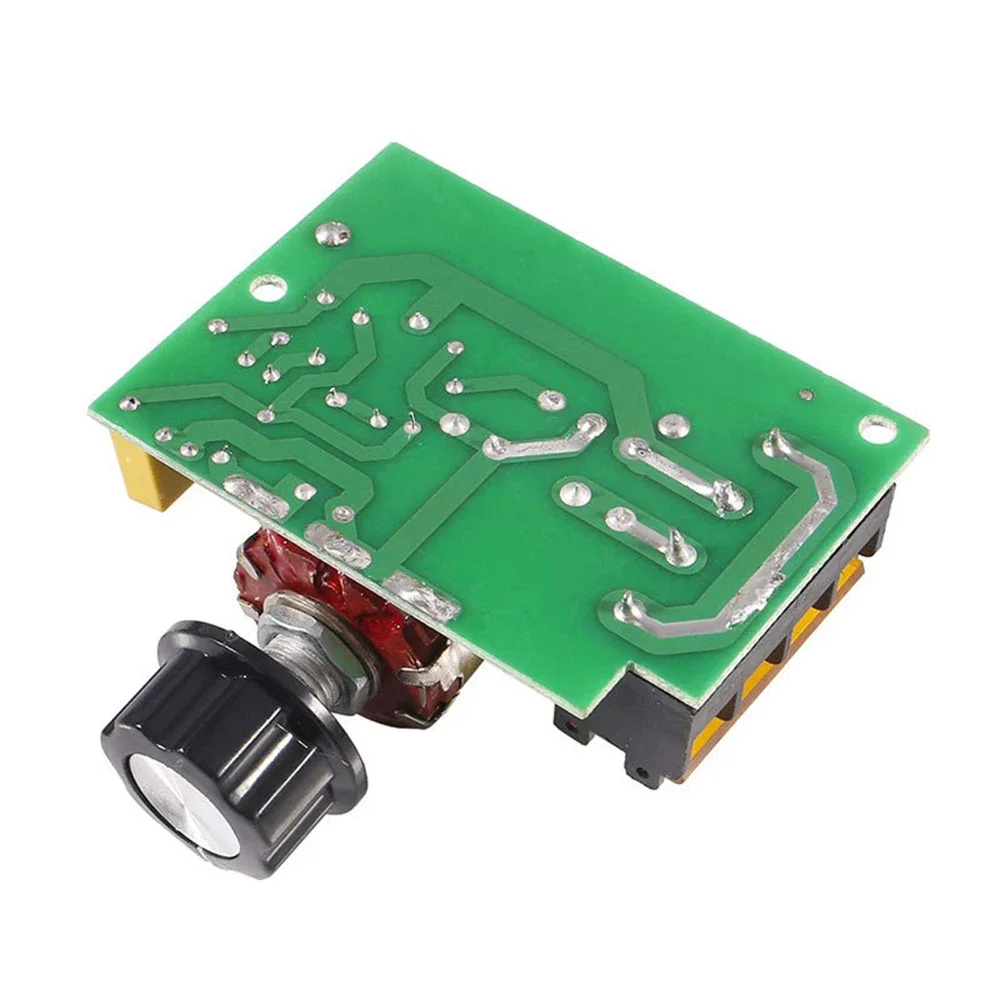This photo showcases a compact, green circuit board set against a white, featureless background. The board is rectangular with a distinctive 90-degree notch cut out of the bottom right corner and two holes drilled at the top right and center left for mounting. Various colors on the board include green, silver, gray, yellow, red, and black, creating a vivid contrast. The board features soldered circuitry and raised components, such as angled channels and pins soldered at specific points, likely to secure connections. Notably, the bottom left of the board houses a prominent black knob or dial, which appears to be adjustable, suggesting it might control different functions of the board. A gray part resides on the right side, and a yellow stand supports the other side, with a red component visible beneath. The detailed and colorful circuit board implies it's a part of a larger electronic equipment setup, potentially being sold as a standalone component.